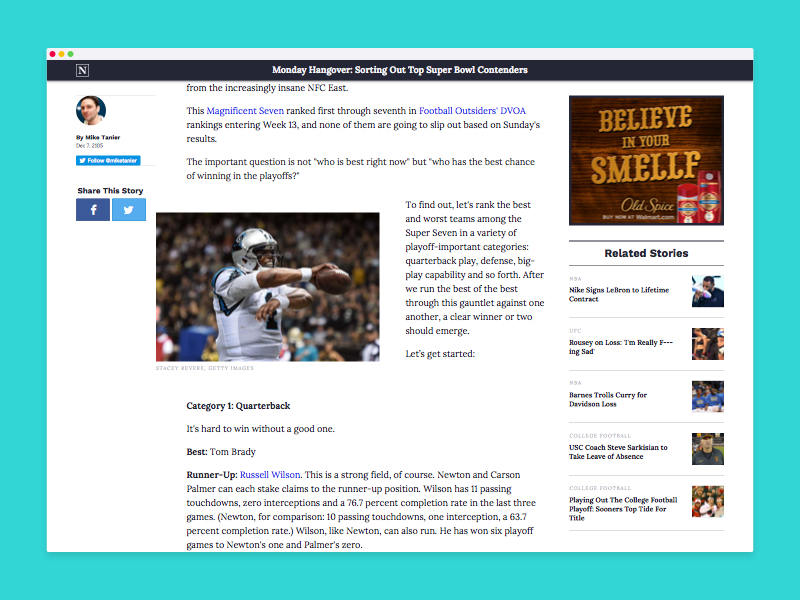Screenshot of a web page viewed on a laptop or desktop computer, featuring a rectangular, teal border framing a white content area. At the top of the webpage, classic Apple window control icons—red, yellow, and green dots—are visible. Below the window controls, a long black navigation bar with white text features an 'N' logo inside a white box on the left and a headline that reads "Monday Hangover: Sorting Out the Top Super Bowl Contenders."

The article is authored by a man with dark hair, wearing a blue shirt, set against a blue background, though his full name is partially obscured. The main section of the screenshot includes an image of football player Cam Newton, centered towards the left, holding a football in his right hand, with text below identifying him as "Category 1 Quarterback."

On the right side, an advertisement is displayed in a brown box with yellow-orange lettering that reads "Believe in Your Smelf," accompanied by two images of deodorant. Below the ad, a column titled "Related Stories" lists five football-related thumbnails, each representing a different article. At the very bottom, social media icons for sharing the story via Facebook or Twitter are present.